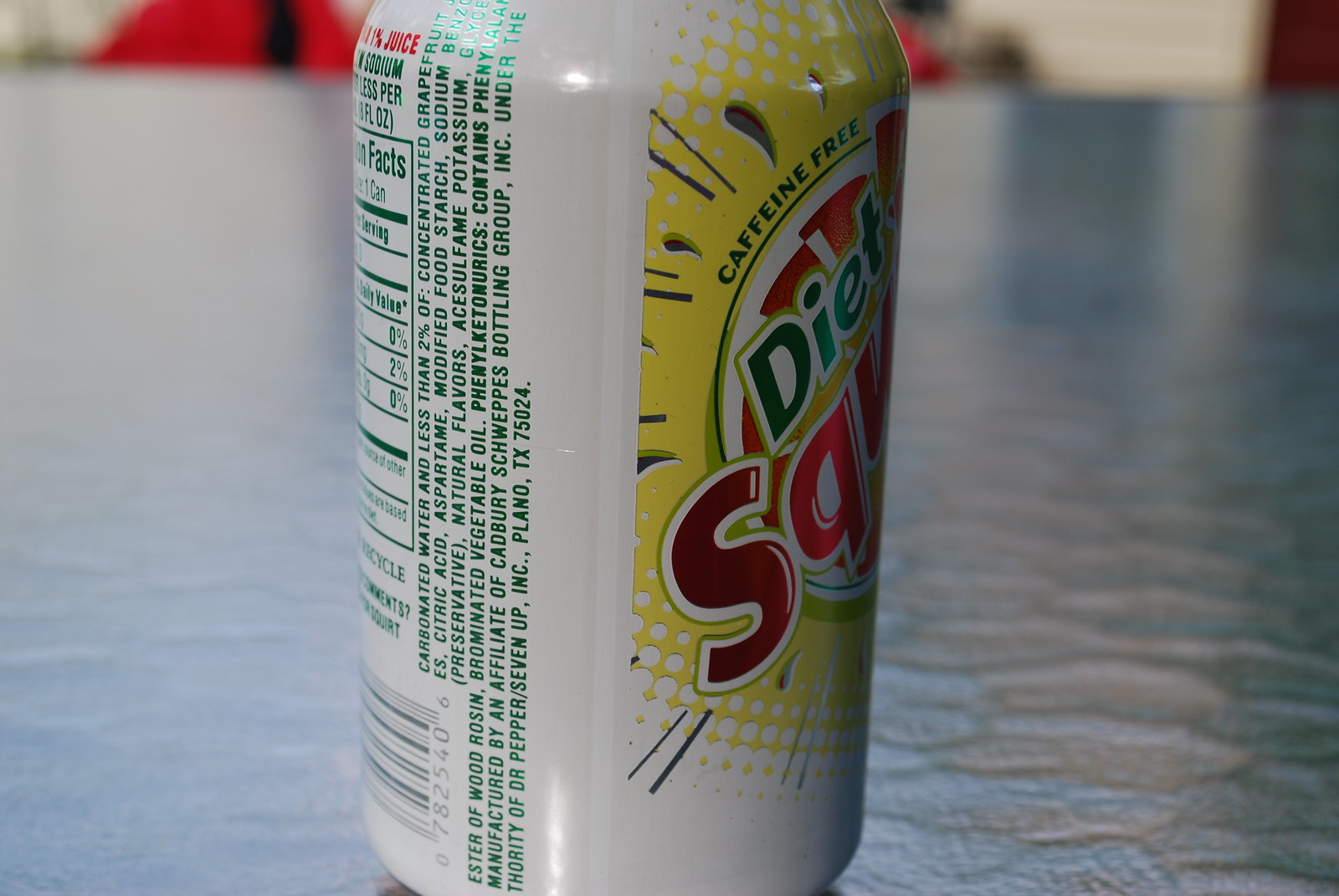The image features a close-up of a can of diet citrus soda, resting on a wavy, blue tabletop. The can's design includes a white base with a noticeable yellow sunburst pattern in the center, interspersed with splashes of green. The front view of the can displays the word "diet" in green lettering and "caffeine-free" above in matching green. A white circle at the center of the sunburst contains the letters "SQ" in red. The left side of the can shows partial nutritional information and a QR code at the bottom, while the ingredients list, written in green, is positioned sideways up the side of the can. The background includes hints of red and black elements and a white wall. The top and bottom edges of the can extend beyond the image frame, emphasizing the central details. The can's overall appearance includes burgundy and green font, and under the ingredient list, it states its packaging by Dr. Pepper 7-Up Inc. in Plano, Texas.